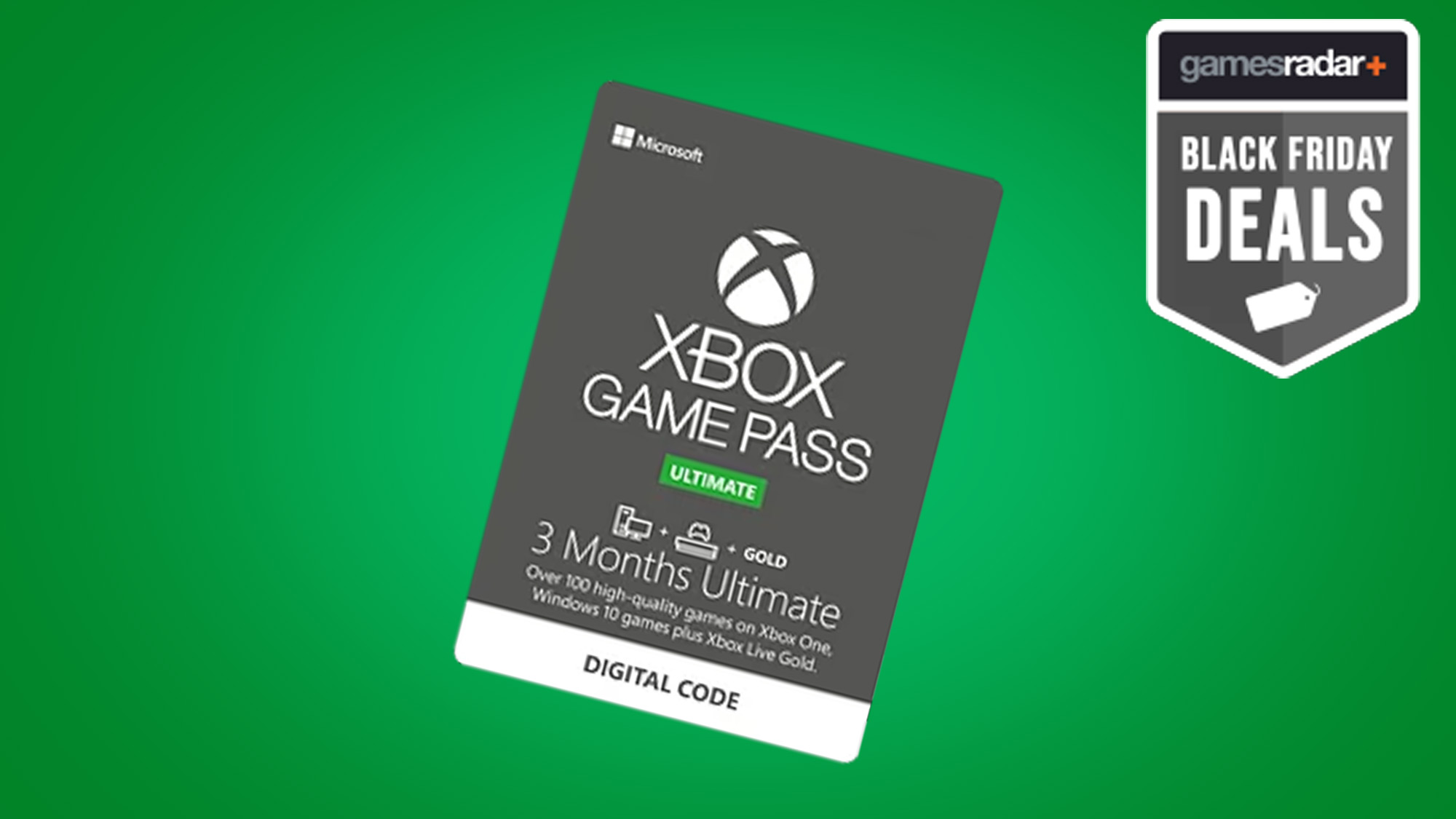The image is an advertisement for a Black Friday deal from a video game company. It features a landscape-oriented composition with a solid green background and a subtle circular gradient in the center, making that area slightly lighter. 

In the upper right-hand corner, there's a pentagonal shape outlined in white. This shape is split into two sections; the top section is rectangular and contains the text "Games Radar," while the bottom section, also outlined in white, displays "BLACK FRIDAY DEALS" in capital letters, with "Deals" being the largest and boldest part of the text. Additionally, a small tag icon accompanies this text.

Centered on the green background, there is an obliquely rotated rectangle featuring an Xbox Game Pass. At the top of this rectangle, the Xbox logo is prominently displayed, followed by the Microsoft logo in the upper left corner. Below, the text "Game Pass" is inscribed, and beneath this, a green rectangular banner reads "Ultimate." The advertisement emphasizes a three-month subscription to Xbox Game Pass Ultimate, which offers access to over 100 high-quality games across Xbox One, Windows 10, and includes Xbox Live Gold.

Towards the bottom of this central rectangle, the text "Digital Code" informs the viewer that purchasing this deal will provide a digital code for redemption. The advertisement is visually appealing and informative, making it suitable for platforms such as Facebook, webpages, and other social media channels.